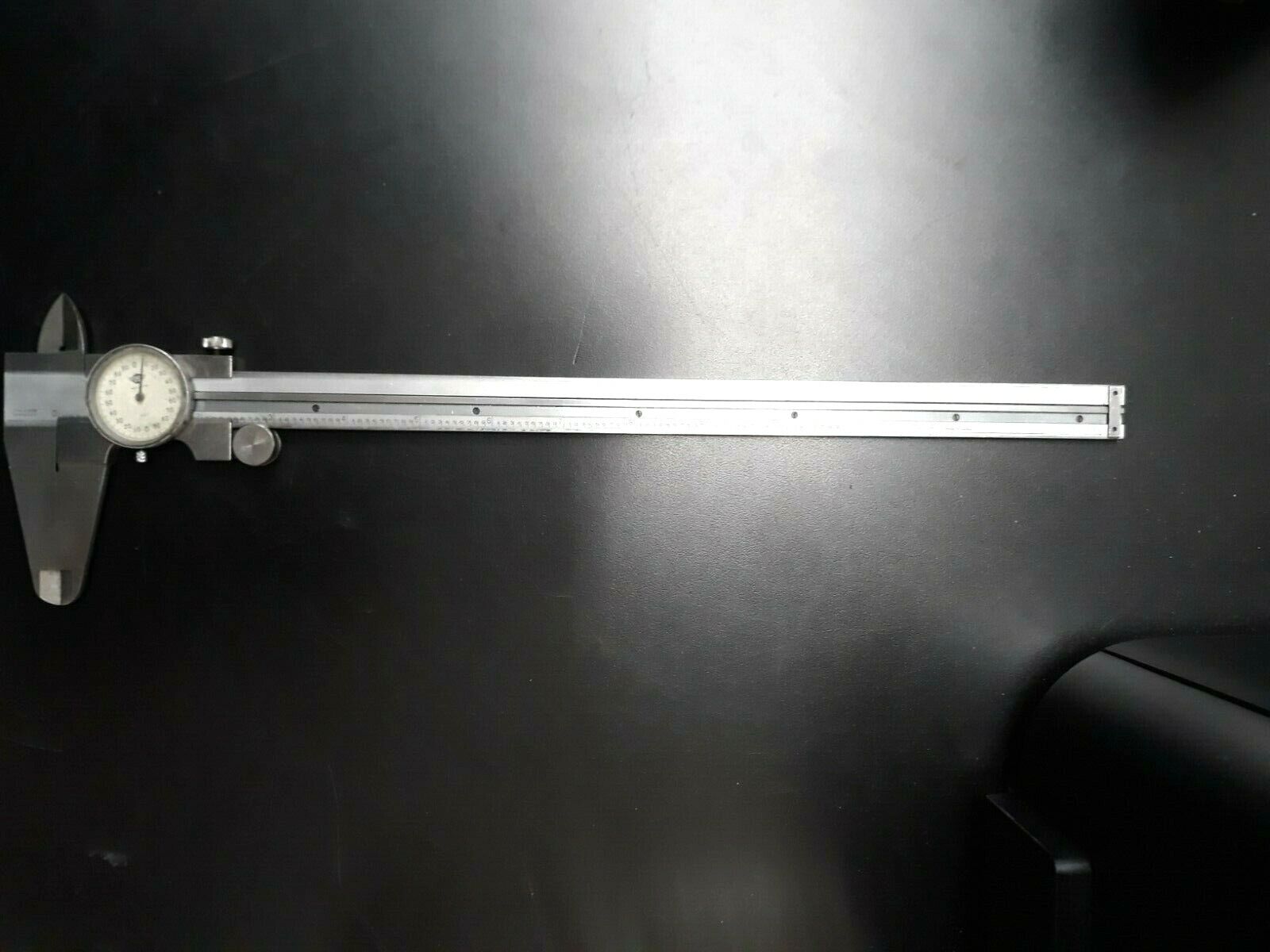The photograph, captured in an indoor setting, showcases a precision measurement tool, likely a caliper, laid horizontally on a shiny black surface. The focal point of the image is a long, silver metallic rectangular bar extending from left to right, adorned with faint measurement markings akin to those on a ruler or tape measure. To the left of this bar is a prominent circular dial resembling a clock face with a silver frame and white background, marked with numbers around its circumference and a single black needle. This dial likely serves as a pressure gauge or diameter indicator. At the far left end, the caliper's clamps are visible, featuring two large metal clamps at the bottom and two smaller ones at the top, suggesting their use for measuring the width or diameter of objects. The image appears slightly overexposed, making some details difficult to discern, yet the essential components – the caliper, the ruler, and the gauge – remain clear. The presence of a black, round-edged object on the bottom right corner adds to the composition, likely serving as part of the tool's base or an accessory.